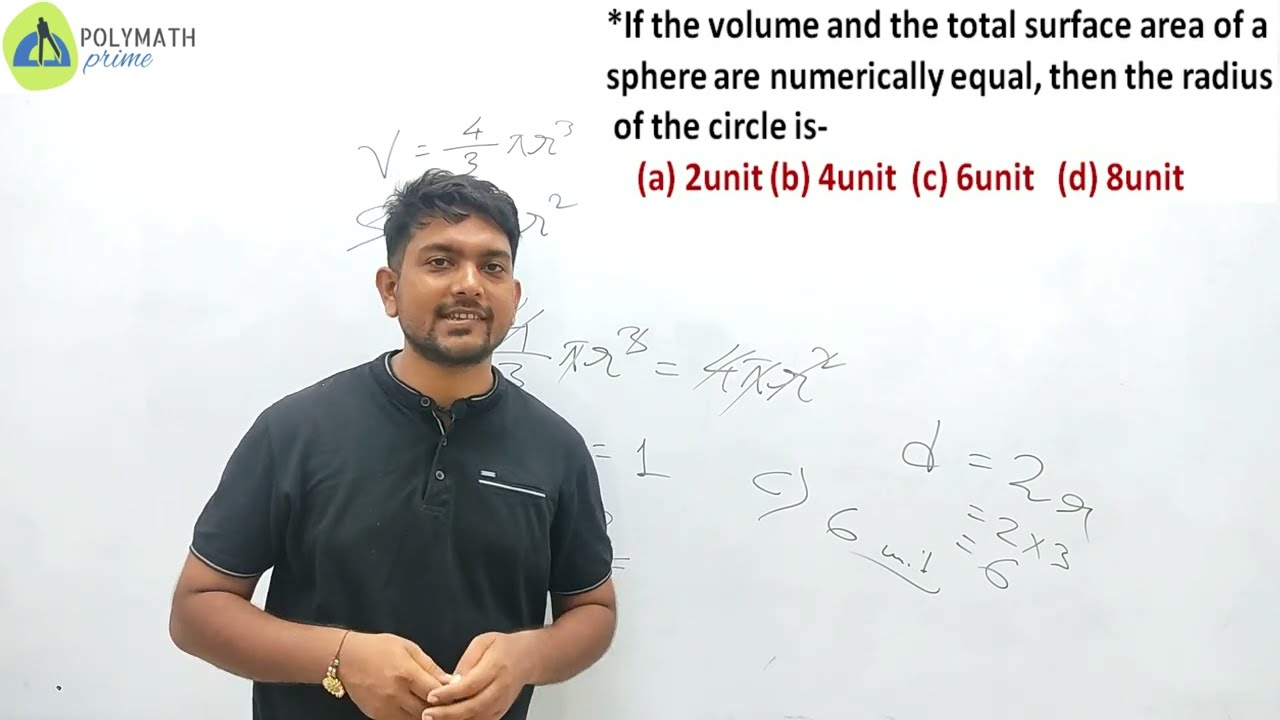The image features a gentleman of Middle Eastern descent, characterized by his tawny brown skin, dark brown medium-length hair trimmed neatly around his forehead, and a slight mustache and beard. He is dressed in a black polo shirt and accessorized with a small gold watch. He is standing in front of a large whiteboard filled with mathematical equations written in black marker, which includes various Greek letters and stretches across five to six rows vertically and trails off horizontally. The equations appear to be related to the volume and surface area of a sphere, but a portion is obscured by his presence. Above the whiteboard, the text “Polymath Prime” is visible in the upper left corner, accompanied by a green and blue logo. Additionally, there is a caption on the screen reading, "If the volume and the total surface area of a sphere are numerically equal, then the radius of the circle is A, 2 unit, B, 4 unit, C, 6 unit, D, 8 unit." This suggests that the image could be a still from an educational video or a screenshot from an online math tutorial.